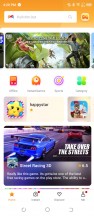The screenshot displays a smartphone interface with a vibrant, colorful layout. The topmost section features a vivid orange header with a white rectangular search bar, flanked by standard smartphone indicators showing the time and battery level. Below the search bar, several clickable colored images are visible, the most prominent one depicting an outdoor landscape with dense green foliage and a whitish sky. An individual in a white shirt and tight black pants stands among the foliage.

Right beneath this outdoor image are four small, circular colored icons, presumably for different categories or functions. Below these icons are four rectangular search options depicted with small square buttons. The first button features a yellow star with a cartoonish face and black eyes over a purple-bordered window with a jagged edge and a blue center. Its adjacent button is gray with a central image of what looks like a Roman soldier, identifiable by red helmet tufts, a red cloak, an armored chest plate, and a helmet.

Further down, there is a large, rectangular image of two cars racing, captured from a rear perspective. The cars, one blue and one red, race on a gray asphalt street under the bold white text, "Take over the streets." Below this image, there is a small game icon with a description in white text.

A rainbow-colored line separates this section from the one below, which contains four separate icons. At the very bottom, three faint gray icons, likely standard smartphone icons, can be seen. The overall interface has a primarily white background, making the colorful images and icons stand out despite the slight blur.